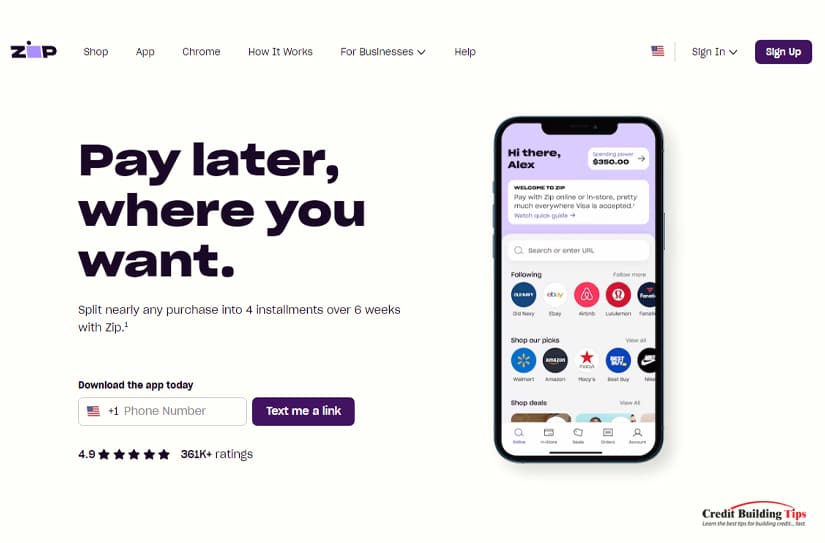In the image depicting a page about the Buy Now, Pay Later service Zip, prominent features are meticulously arranged. In the top-left corner, the familiar Zip logo stands out. The header stretches horizontally across the top, listing options such as "Shop," "App," "Chrome," "How it Works," and "For Businesses," some of which have a drop-down arrow indicating further sub-menu options. Additional menu items "Help," an American flag icon, "Sign In," and a "Sign Up" button complete the header in the top right corner.

Dominating the left side, a bold and large-text proclamation reads, "Pay Later Where You Want." This is followed by a brief description, "Split nearly any purchase into four installments over six weeks with Zip. Download the app today." Directly below, there is a rectangular input box featuring an American flag icon and "+1" code placeholder beside a field labeled "Phone Number." Adjacent to this input box, a button labeled "Text Me a Link" is featured. Below this section, user feedback is showcased with a rating of 4.9 stars, accompanied by an image of five nearly completely filled stars and an assertion of "361k+ ratings."

On the right side, a visual of a smartphone screen captures attention. At the top of the screen within the image, the message "Hi There Alex" is visible, though the subsequent text blur impedes clear readability. Notably, a bolded figure "$350.00" is discernable, along with a welcome text stating, "Welcome to Zip. Pay with Zip online or in-store. Pretty much everywhere Visa is accepted." A call-to-action link, "Watch Quick Guide," is present below this text. Icons representing popular retailers, including Old Navy, eBay, Walmart, Amazon, and Macy's, are displayed beneath the app imagery. Concluding the page, a bottom-right corner note reads "Credit Building Tips."